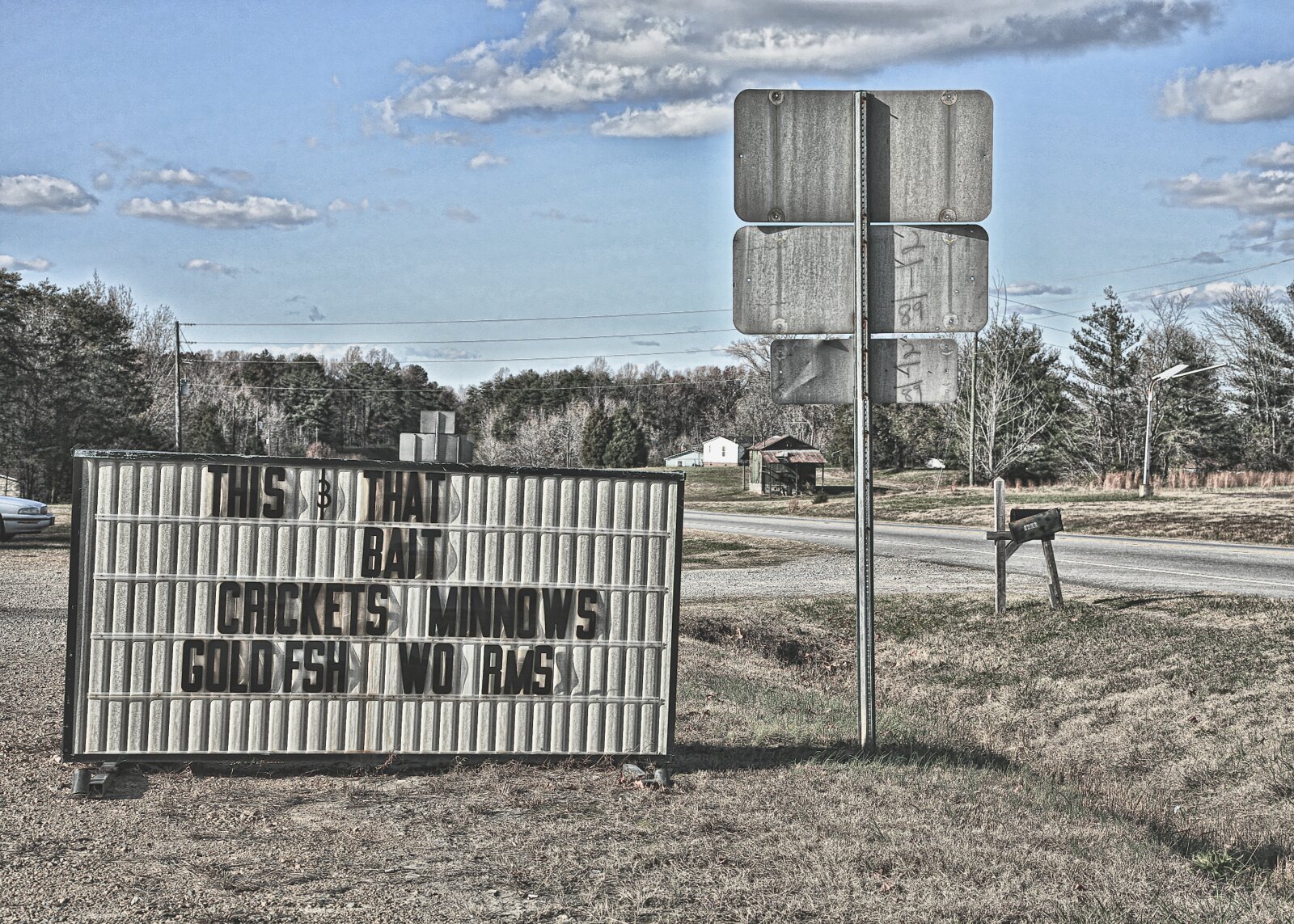In this outdoor daytime photograph, the overarching aesthetic is one of subdued, washed-out colors. The pale blue sky, accentuated with a few white clouds, forms the backdrop. There's a row of greenish-gray trees in the background, while the foreground is dotted with greenish-brown grass, adding to the muted palette.

Dominating the left-hand side of the image is a rectangular marquee sign, resting directly on the ground. The sign is adorned with black letters spelling out a list of items: "this and that, bait, crickets, minnows, goldfish, worms." Adjacent to this marquee on the right stands a narrow, gray metal pole driven vertically into the earth. Mounted on this pole are three signs arranged one below the other, their backs turned to the viewer. The top two signs are rectangles with rounded edges, while the smaller rectangular sign at the bottom completes the array. All that can be seen of these signs are their silvery backsides, reflecting the subdued tones of their surroundings.